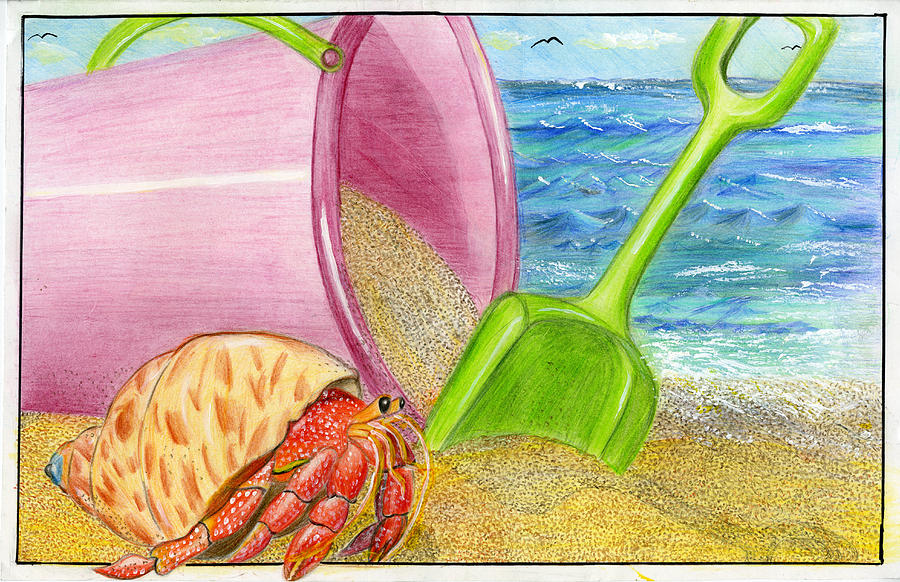The image depicts a detailed and vibrant artistic impression of a serene beach scene, rendered in what appears to be watercolor or pencil crayon. The central focus is on a large, pink plastic bucket tipped over on its side with sand spilling out, accompanied by a bright lime green plastic shovel intended for playful activities like building sandcastles. In the foreground, there is a striking red hermit crab with stalk-like yellow eyes ending in black dots, visible claws, and carrying a conch shell on its back, wandering near the bucket and shovel. The background captures the essence of a peaceful shore, showcasing ocean waves with gentle ripples under a blue sky dotted with white clouds. Black-outlined seagulls soar through the sky, enhancing the natural ambiance of the scene.